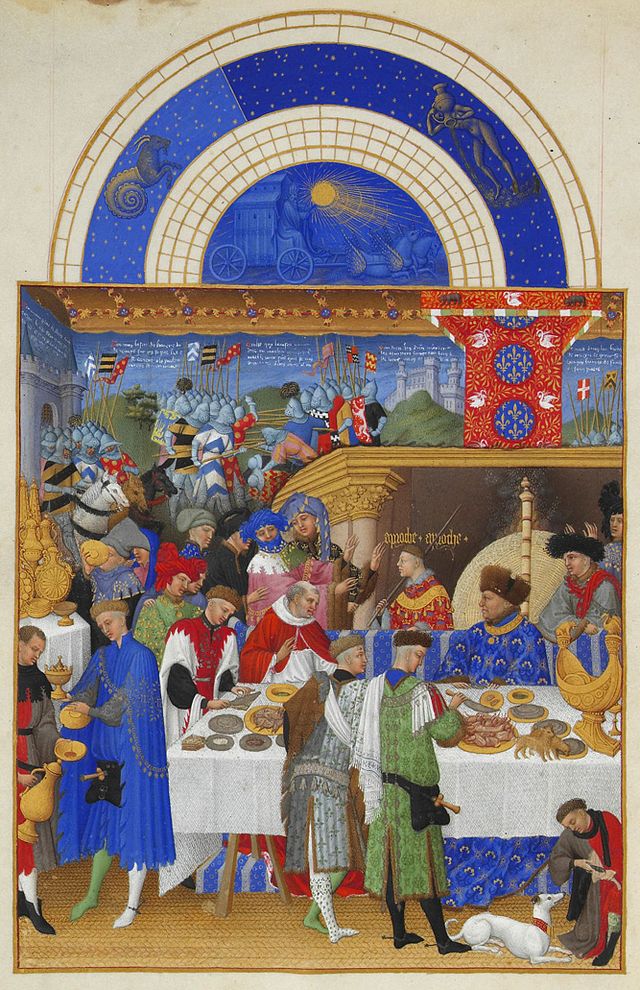This large and detailed medieval painting vividly illustrates a grand, festive banquet. In the foreground, a group of clergymen and royalty are gathered around a lavish table adorned with various types of food. Some figures are dressed in ornate Catholic vestments, including red and white robes, enhancing the scene's religious undertone. A white dog is seen in the bottom right corner, eagerly begging for scraps. To the right, animals are depicted eating the food laid out, which adds to the lively atmosphere. In the background, there are women wearing headscarves, possibly indicating their noble or royal status. Beyond them, a dramatic scene unfolds, featuring knights in metal armor and helmets engaged in battle, carrying clan flags that add to the historic ambiance. Above it all, an arch painted with celestial imagery and stars crowns the scene, adding a sense of grandeur and otherworldliness. The vibrant palette includes reds, oranges, blues, purplish pinks, gold, greens, grays, blacks, beige, and silver, all meticulously applied to enhance the painting's intricate details.